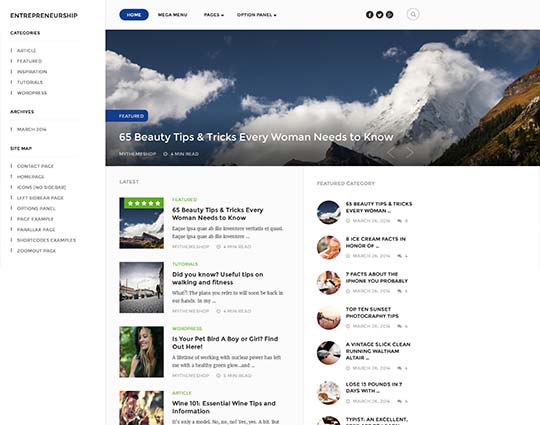This screenshot captures a lifestyle website geared towards women, showcasing a range of articles and tips relevant to their interests. The website features a clean, predominantly white background with a well-organized layout.

On the left-hand side, there is a vertical menu bar with the word "Entrepreneurship" prominently displayed in black text at the top left corner. Below, several categories such as "Categories," "Archives," and "Site Map" are listed, suggesting a comprehensive and easy-to-navigate structure typical of a magazine or publication website.

Centered at the top, there is a horizontal navigation menu with the "Home" tab highlighted in a blue circle with white text, indicating that it is the active page. Adjacent to it are tabs labeled "Mega Menu," "Pages," and "Option Panel," denoting different sections of the site. The top right corner features icons for Facebook, Twitter, and Pinterest, offering direct links to the website's social media channels, alongside a magnifying glass icon for search functionality.

The main content area displays a featured section prominently, with an image of a mountainous landscape shrouded in clouds. Overlaid text reads "Featured: 65 Beauty Tips and Tricks Every Woman Needs to Know," linking to what appears to be a key article. Below, the content is organized into two vertical columns, featuring various articles such as "Eat Ice Cream: Facts in Honor of..." and "Top 10 Sunset Photography Tips," each serving as links to further detailed posts on these topics.

Overall, the structured design and diverse content suggest this is a dynamic and resourceful website tailored to women's lifestyle needs.